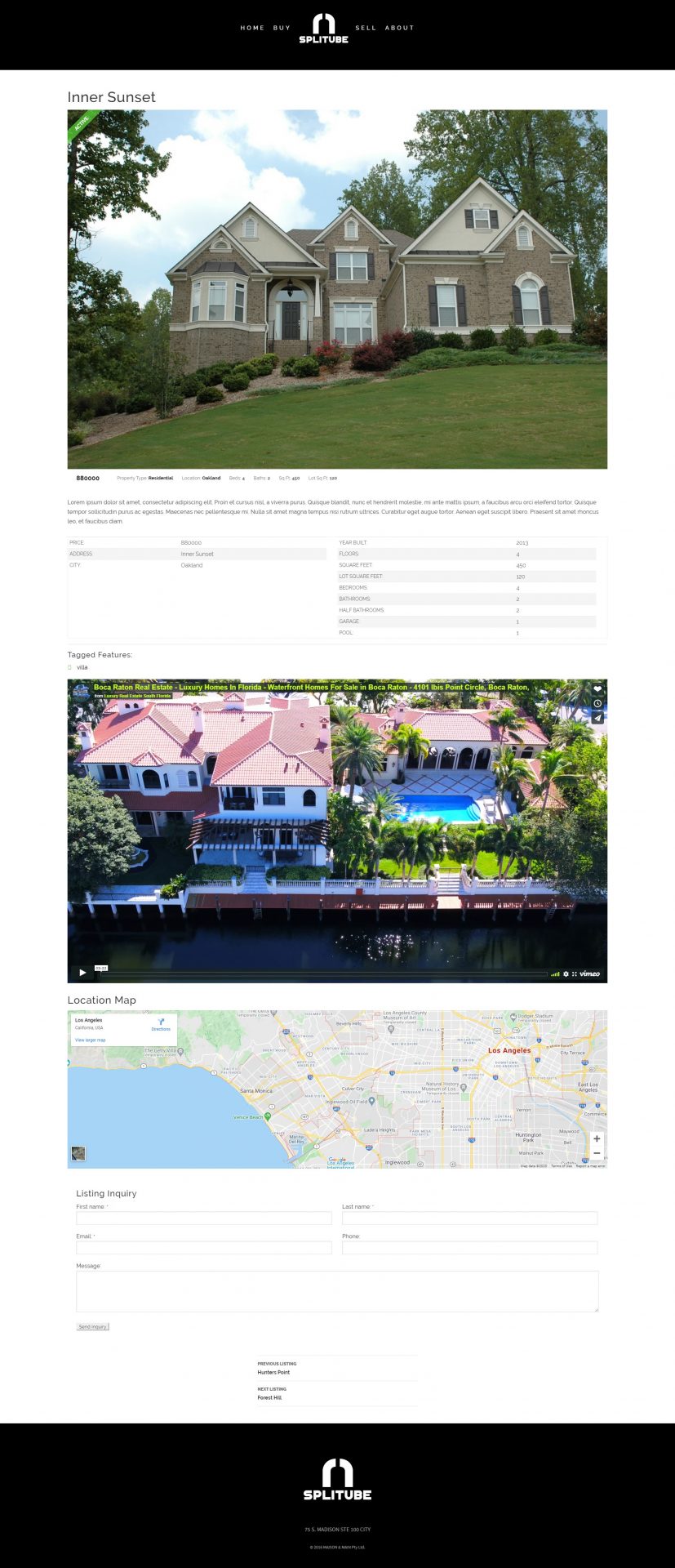**Web Page for a Real Estate Listing: "Simple Tube"**

**Header:**
At the very top, there's a black header featuring the Simple Tube logo centered in white, which resembles a stylized "S" that evokes the shape of a building or an archway. To the right of the logo, navigation links are horizontally aligned, including "Buy," "Sell," and "About."

**Main Content:**
The main page's title is "Inner Sunset" in large, bold text.

**Primary Image:**
The top image showcases a traditional, large two-story house with a manicured lawn. The house features a combination of brick and light-colored siding, several windows with white frames, and a centrally located front door with a covered porch. The well-kept lawn, shrubs, and small plants line the front of the house.

**Property Details:**
- **Location:** Oakland
- **Type:** Residential (tagged as a villa)
- **Bedrooms:** 4
- **Bathrooms:** 2
- **Square Footage:** House - 450 sq. ft., Lot - 320 sq. ft.

**Secondary Image:**
The next image highlights a luxurious property likely located in Florida. This property features multiple buildings with red tile roofs, a backyard with a large swimming pool, and lush greenery including palm trees. The property is adjacent to a body of water, possibly a canal or a lake.

**Map Image:**
A map follows, highlighting the location of the property, showing a section of Los Angeles as well as various other landmarks around the U.S.